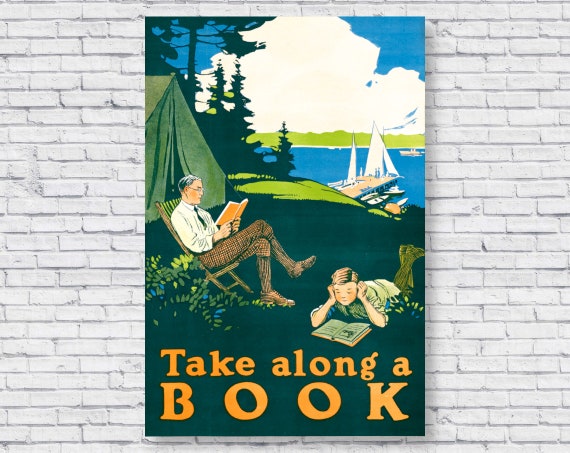In the center of a white brick wall hangs a vertically-oriented portrait-style illustration that immediately captures attention with its scenic camping site depiction. The detailed image showcases a peaceful lakeside setting against a backdrop of green hills and a vibrant blue sky filled with large, fluffy white clouds. 

In the immediate foreground, a father sits comfortably in a folding chair, reading an orange book. He is dressed in a white dress shirt, a tie, and checkered brown pants. By his side, a young boy lounges on his stomach in the lightly grassy terrain, also absorbed in a book, his legs kicked up behind him. Their campsite is completed with a green tent positioned in the upper left area of the illustration, amid sparse tree coverage.

Further in the background, a serene lake stretches out, dotted with a pier and several boats, enhancing the tranquil vibe of the scene. Across the bottom of the illustration, in bright orange text, reads the phrase: "Take along a book."

The colors within the illustration are harmonious, with varying shades of green, blue, brown, and touches of yellow and orange, creating a vivid and inviting atmosphere that emphasizes the joy and calmness of a rustic camping retreat.